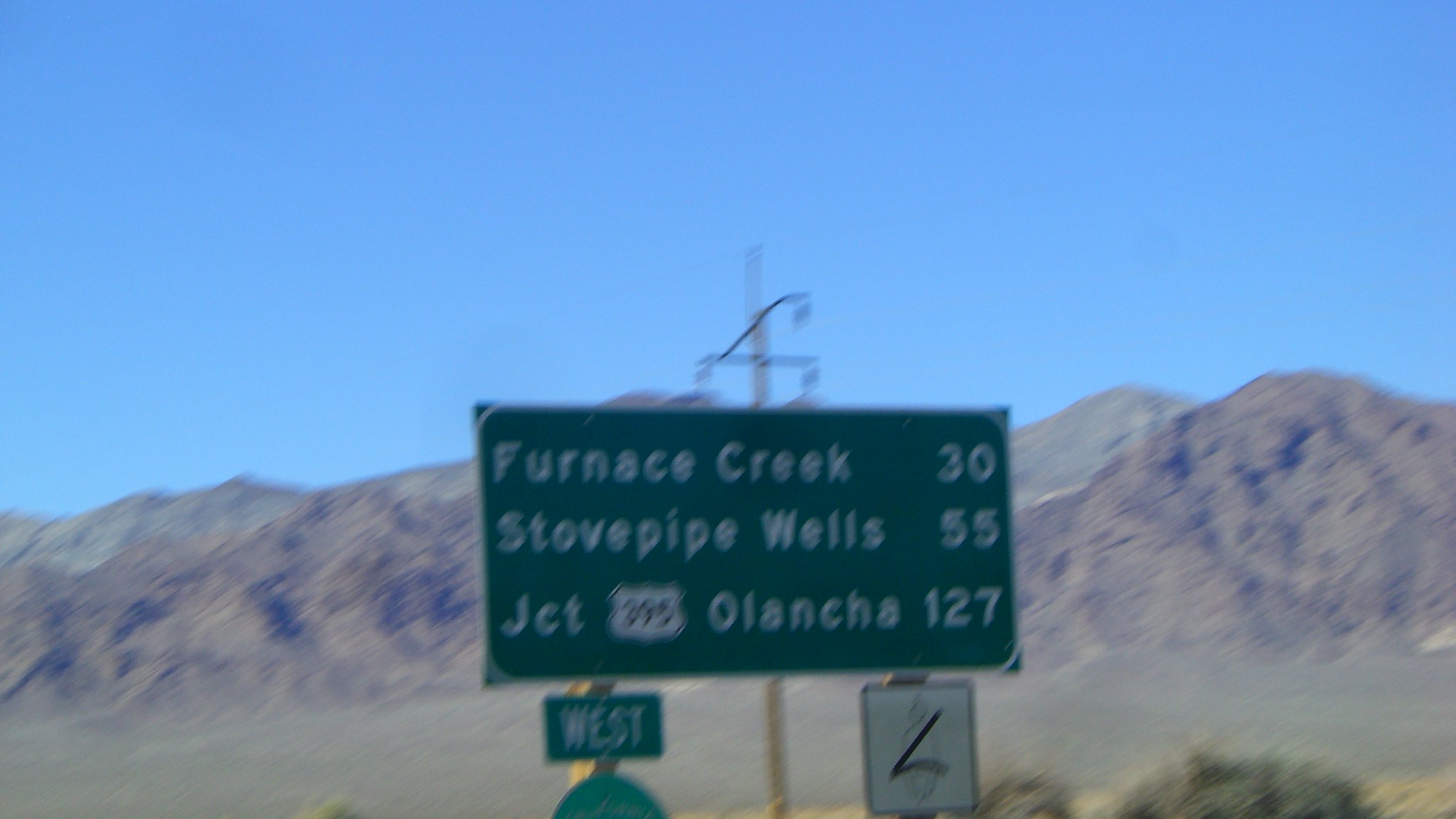This horizontally oriented color photograph captures a blurred street sign on the side of a road, likely taken from inside a moving car. The green sign, positioned centrally in the image, is shadowed but predominantly green in color. It lists three destinations in white text: "Furnace Creek 30," "Stovepipe Wells 55," and "Junction 395, Olantcha 127," with their respective distances. Below the left side of the larger sign, a small green rectangle reads "West." On the right side, a white sign displays an inverted number "7." In the background, rocky foothills stretch out under a medium sky blue sky, adding to the depth and setting of the scene.